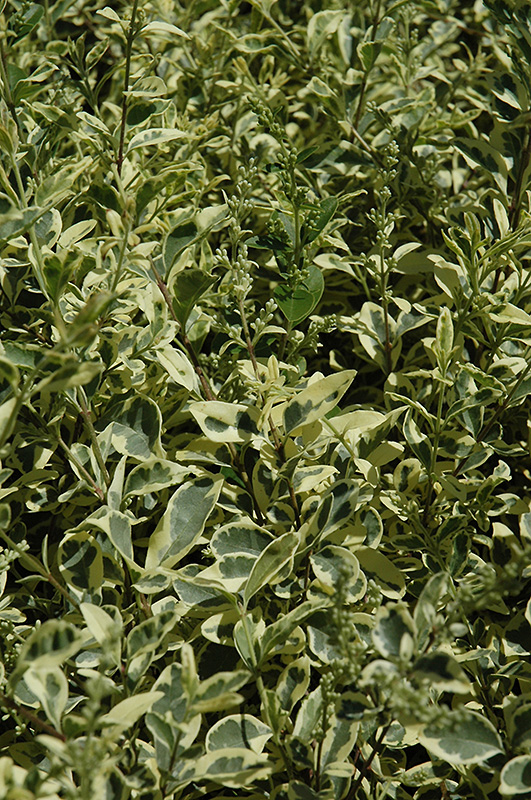The vertical image captures a dense outdoor area filled with overgrown plants, primarily composed of stems and leaves of various shades of green and yellow. The pale green stems, some tinged with yellow and darker green hues, support leaves that are oval-shaped and display distinctive two-toned patterns. The leaves feature pale yellow edges with darker green centers, creating a striking contrast. Small berries or flower buds appear at the tips of some stems, adding subtle details to the foliage. The background and some leaves in the foreground appear slightly out of focus, emphasizing the center leaves that are sharp and detailed. Among the plants, there seems to be a second species with uniformly green leaves. Sunlight casts shadows and reflections on the leaves, indicating it is a sunny day. The image predominantly showcases the lush, varied textures and colors of the leaves, giving it a rich, natural appearance.